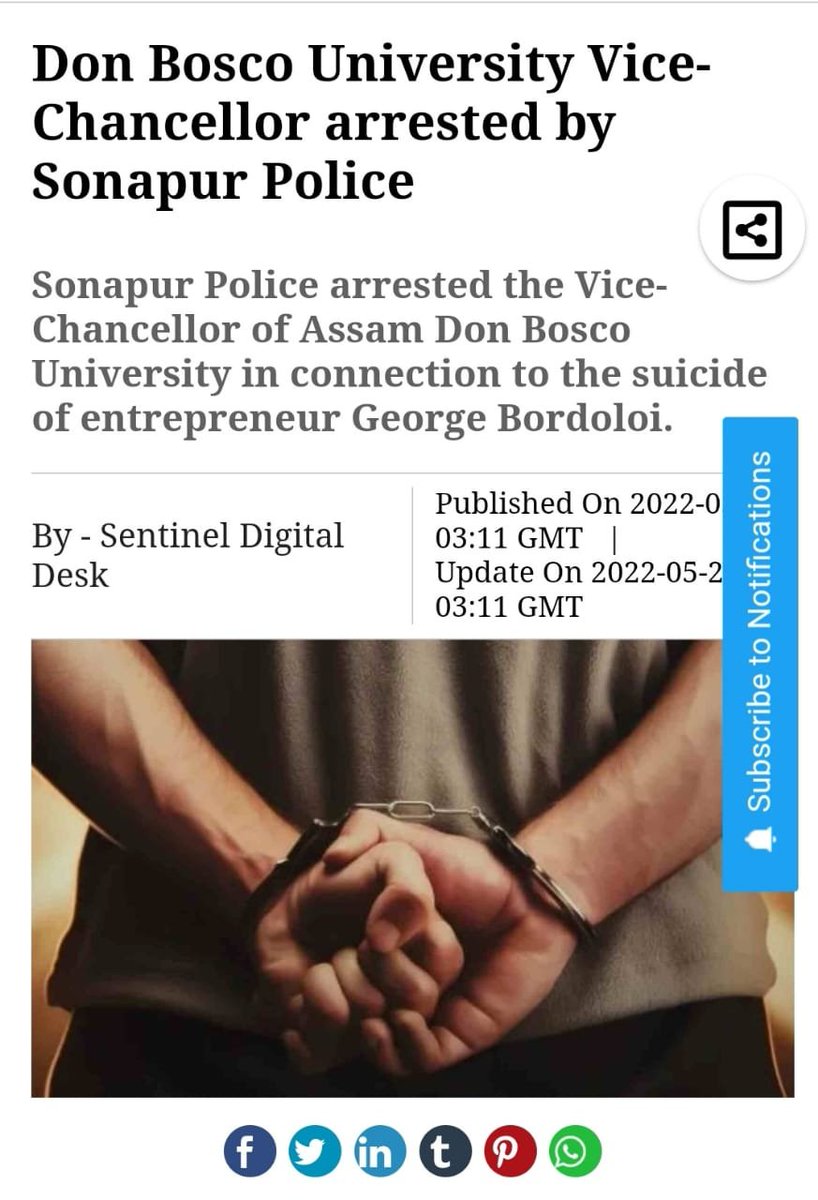Caption: 

A screenshot from the Sentinel Digital Desk features an article titled "Don Bosco University Vice Chancellor Arrested by Sonapur Police". The subheading reveals that the Vice Chancellor of Assam Don Bosco University was arrested in connection to the suicide of entrepreneur Gregor Bordoloi. Authored by the Sentinel Digital Desk, the article includes a publishing date and time partially obscured by a blue notification banner with a bell icon and the text “subscribe to notifications.” The visible portions of the date and time indicate the article was published and updated in 2022 at 3:11 GMT. 

The accompanying image shows the back profile of a man with his hands cuffed behind him, clenched into fists. He is dressed in a brownish-gray shirt and black track pants with white stripes on the sides. At the bottom of the screenshot, social media icons for Facebook, Twitter, Indeed, TikTok, Pinterest, and potentially Telegram are visible, allowing readers to share the article across various platforms.